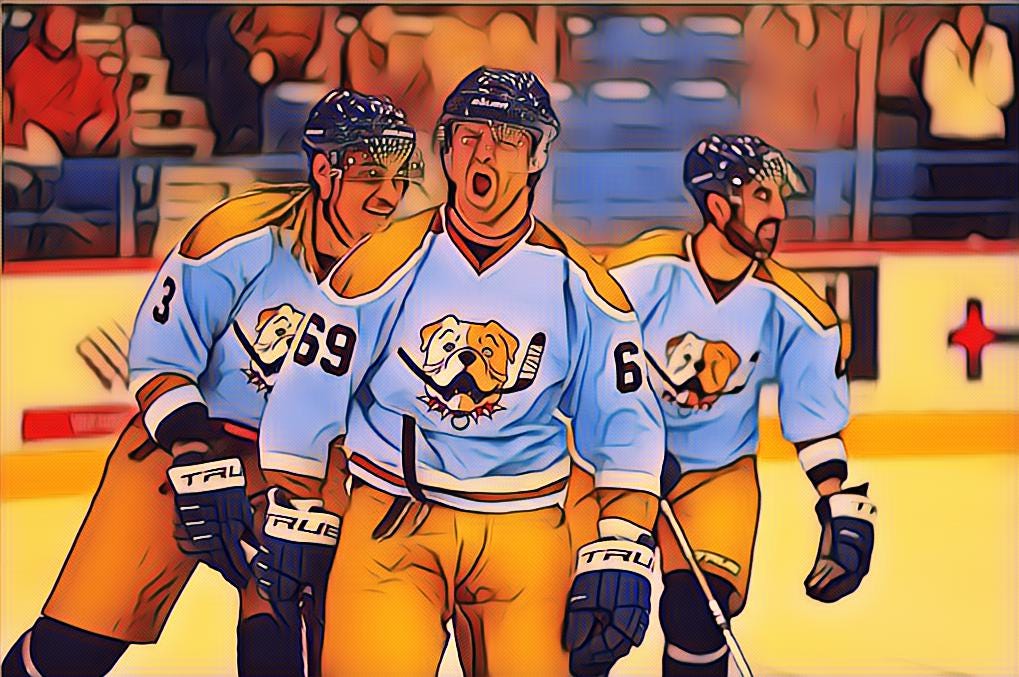In this vibrant and animated digital image, three hockey players sporting a cartoonish style stand prominently in the foreground against the backdrop of a bustling hockey arena filled with faceless spectators donned in jackets, some standing and some seated. The players are all clad in identical uniforms featuring light blue jerseys with gold shoulders, gold shorts, and dark helmets equipped with glass face shields. Their attire is completed with bluish gloves and distinctive gold collars. Central to their jerseys is a striking emblem of a bulldog with a half-tan, half-white face, gripping a broken hockey stick in its mouth and wearing a red spiked collar. The man in the middle, number 69, stands out with his mouth wide open as if yelling, while his two teammates, including a bearded player on his right wearing the number 3, look to their right with smiles. The scene captures the dynamic energy and vibrant spirit of a live hockey game within a comic-inspired setting.